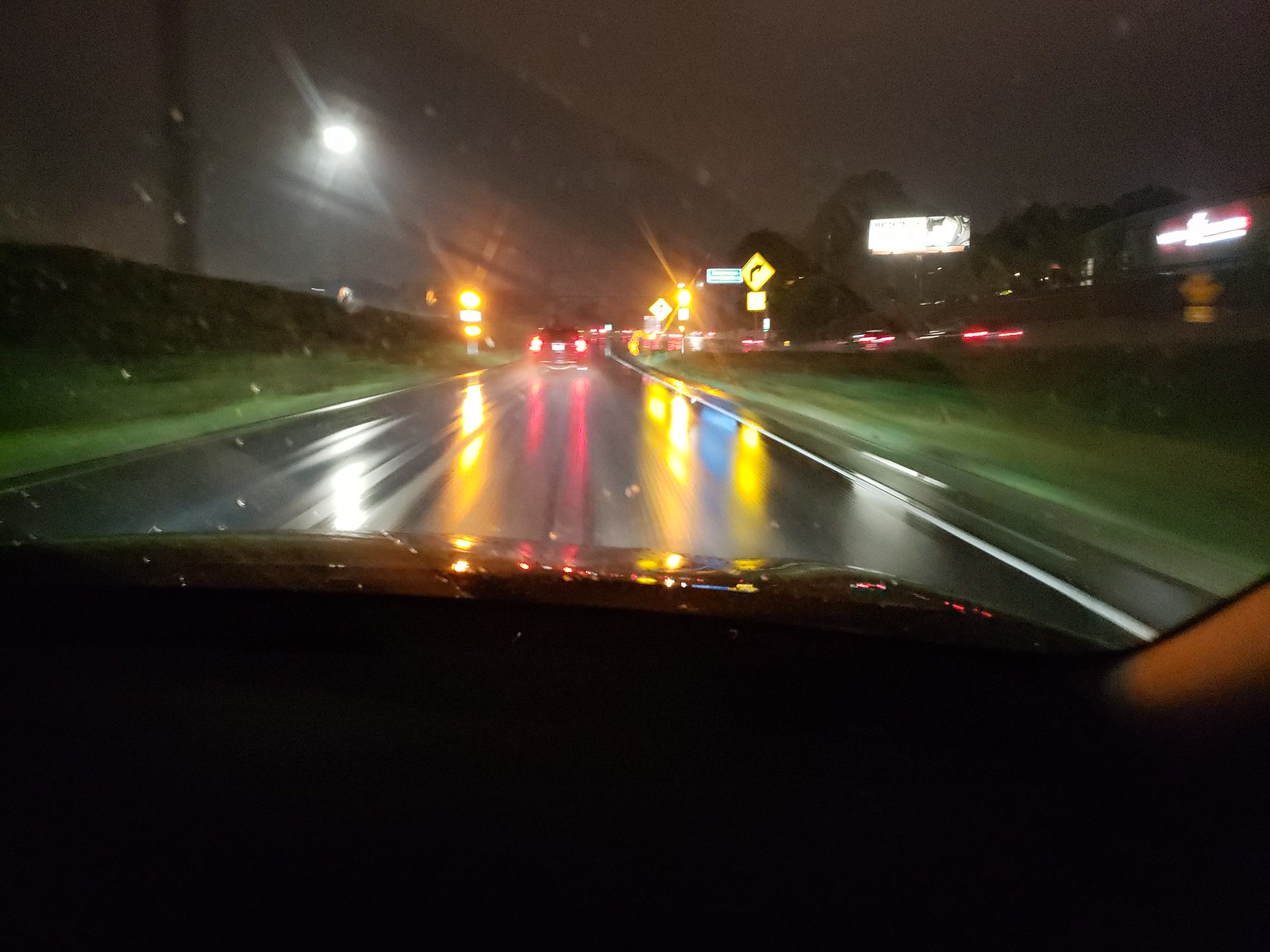The image captures a nighttime scene through the dirty windshield of a car, likely taken while it was raining, evident from the water droplets on the glass and the wet road ahead. The dashboard and hood of the car are visible. To the left of the road, there's a grassy area with a power pole, a wall, and a streetlight farther down. The right side features another grassy area, a lane of traffic with yellow road signs, a yellow fire hydrant, a building, and a billboard backed by a row of trees. The wet highway ahead is blurred with streaks of light from various light sources, including streetlights, street signs, and the taillights of the car in front. A caution sign indicates an upcoming curve, though the suggested speed limit is unreadable. Some clouds are discernible in the dark sky, hinting at the rainy weather despite the limited visibility.